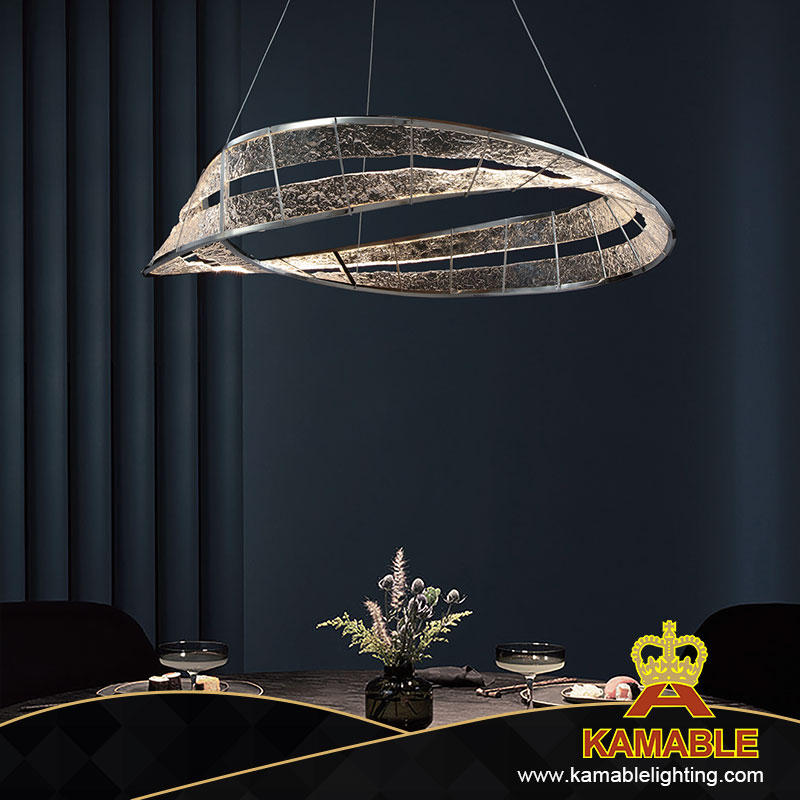This image features a modern, artistic chandelier with a sleek, silver design that closely resembles a Mobius strip, elegantly suspended above a table by three thin wires against a dark, black backdrop with matching curtains. The table below showcases a chic arrangement, including a small gray vase with green, fern-like plants and hints of lavender. Place settings on either side of the arrangement include dark gray plates and unique, flat martini glasses. In the bottom right corner of the image, the text "K-A-M-A-B-L-E" appears with a website URL for Kamable Lighting, accompanied by a logo featuring a crown and a stylized "A" reminiscent of the Eiffel Tower.